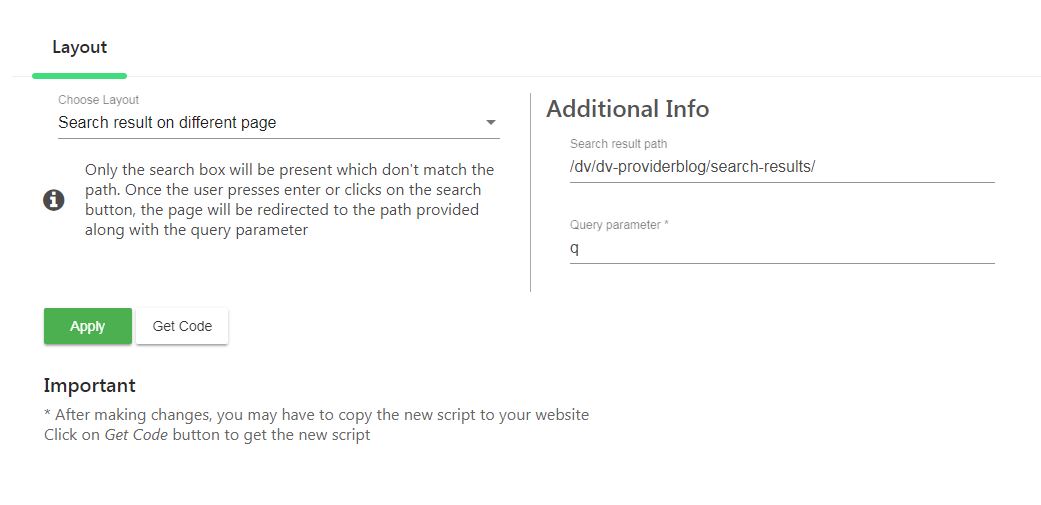Here is a detailed and cleaned-up caption for the image described:

The image features a partial screenshot of a web page focused on layout configuration. At the top, the heading reads "Layout." Directly below, there is an instructional text stating "Choose Layout," accompanied by a drop-down menu. Within the drop-down menu, the selected option is "Search result on different page." Beside this, an information icon is followed by a message explaining, "Only the search box will be present which doesn't match the path. Once the user presses Enter or clicks the search button, the page will be directed to the path provided along with the query parameter."

Further down, the screenshot shows two buttons: a green "Apply" button (indicating it is selected) and a white "Get Code" button. Below these buttons, there is an important message marked with an asterisk: "After making changes, you may have to copy the new script to your website. Click on the Get Code button to obtain the new script."

On the right side of the page, additional information is provided under the heading "Search Results Path." The path displayed is "/dv/dv-provide-blog/search-results/." Beneath this is a field labeled "Query Parameter," which contains the single character "K" on the line.

This detailed caption describes the content and layout of the screenshot, highlighting the key elements and user instructions present on the web page.